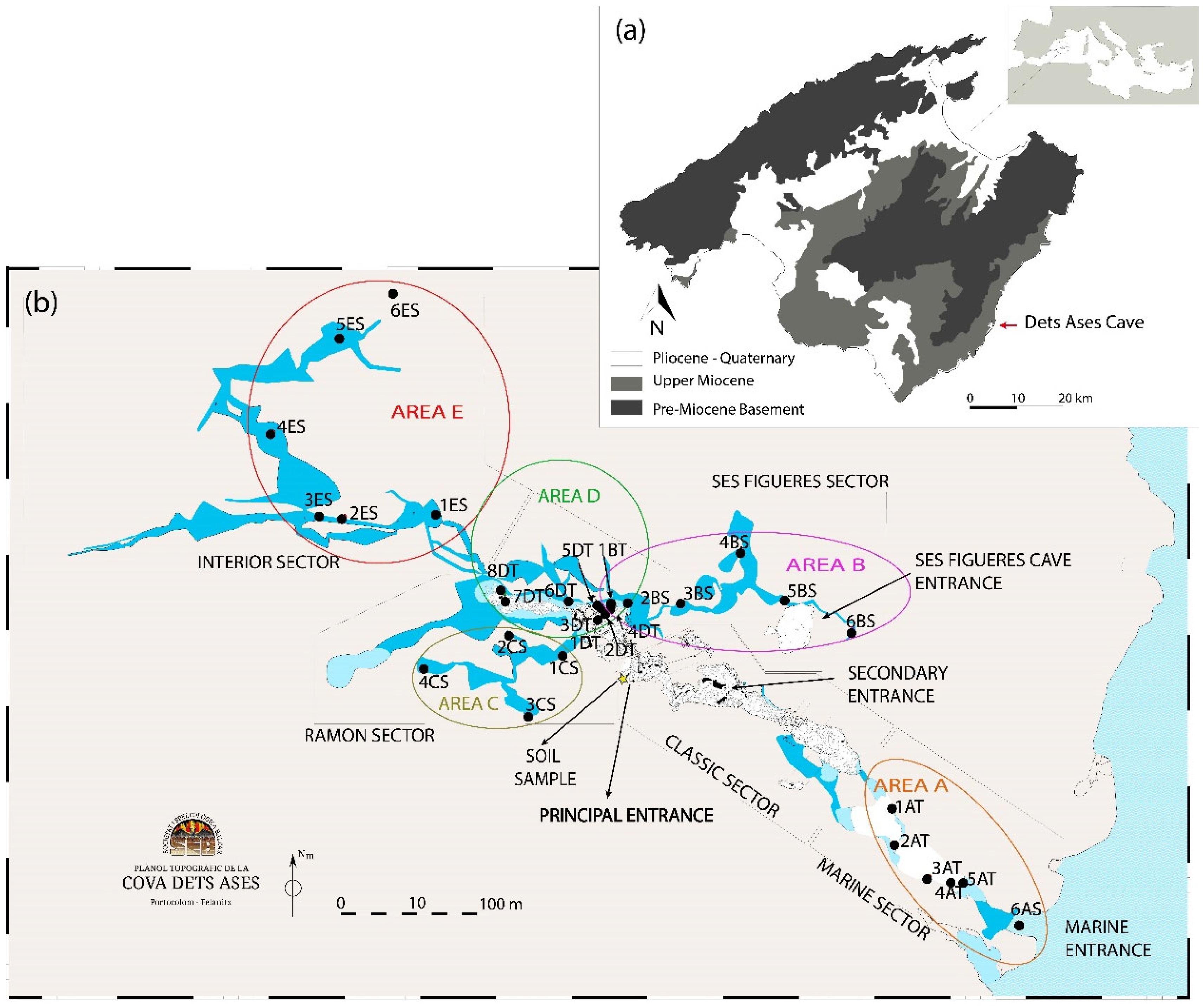This image features two distinct maps, a smaller one positioned in the upper right corner and a larger one below it. Both maps are black and white, but the main map on the bottom includes some gray shaded areas and labeled water bodies like the "Marine Entrance." This larger map, featuring a dashed black line around it, delineates various areas marked as A, B, C, D, and E, with additional labels such as "Interior Sector," "Raymond Sector," "Soil Sample Principal Entrance," and several blue-marked areas. The bottom-left corner of this map showcases a logo that reads "Cova de Ares" in another language.

The top-right map, partially overlapping the lower map, includes a key indicating different geological periods: white for Pielocene Quaternary, gray for Upper Miocene, and black for Pre-Miocene Basement. It also features an arrow pointing to a location labeled "Cova de Ares" along with a scale ranging from 0 to 20 kilometers.